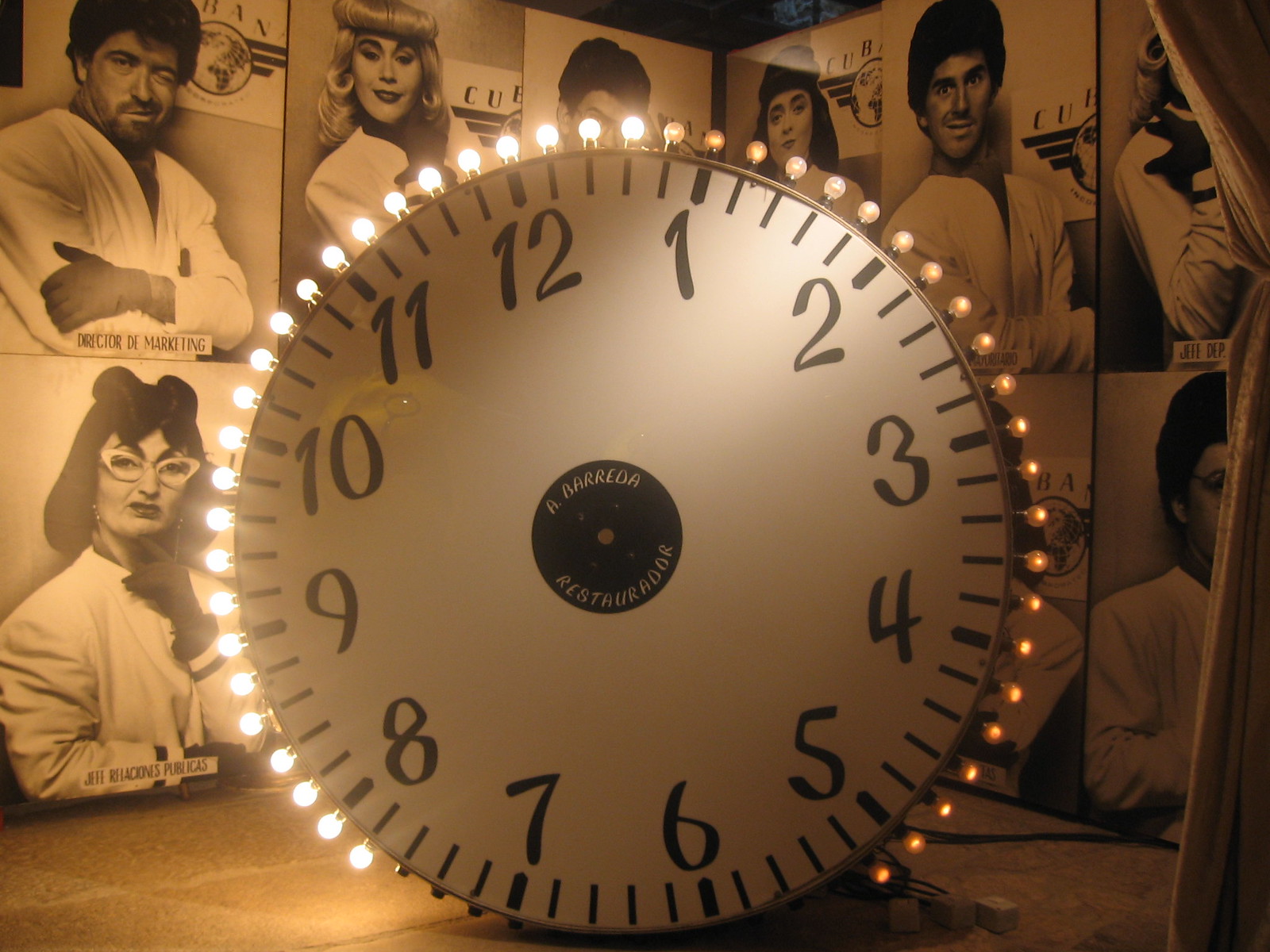The image features a large, white-faced clock with black numbers, tilted slightly to the left so that the number 12 is not perfectly aligned at the top. Encircling the clock are tiny light bulbs that are bright and white on the left side, gradually dimming and turning orange as they progress to the right, with some bulbs completely dark or missing. At the center of the clock is a prominent black circle inscribed with the words "A Bereda Restaurador." The clock is positioned on a brick-like surface of brownish color with gray grout. In the background, there is a panelled wall displaying black and white photographs of various people, who appear to be wearing white shirts and gloves, making different expressions. The majority have dark hair, except for one woman with light-colored hair.